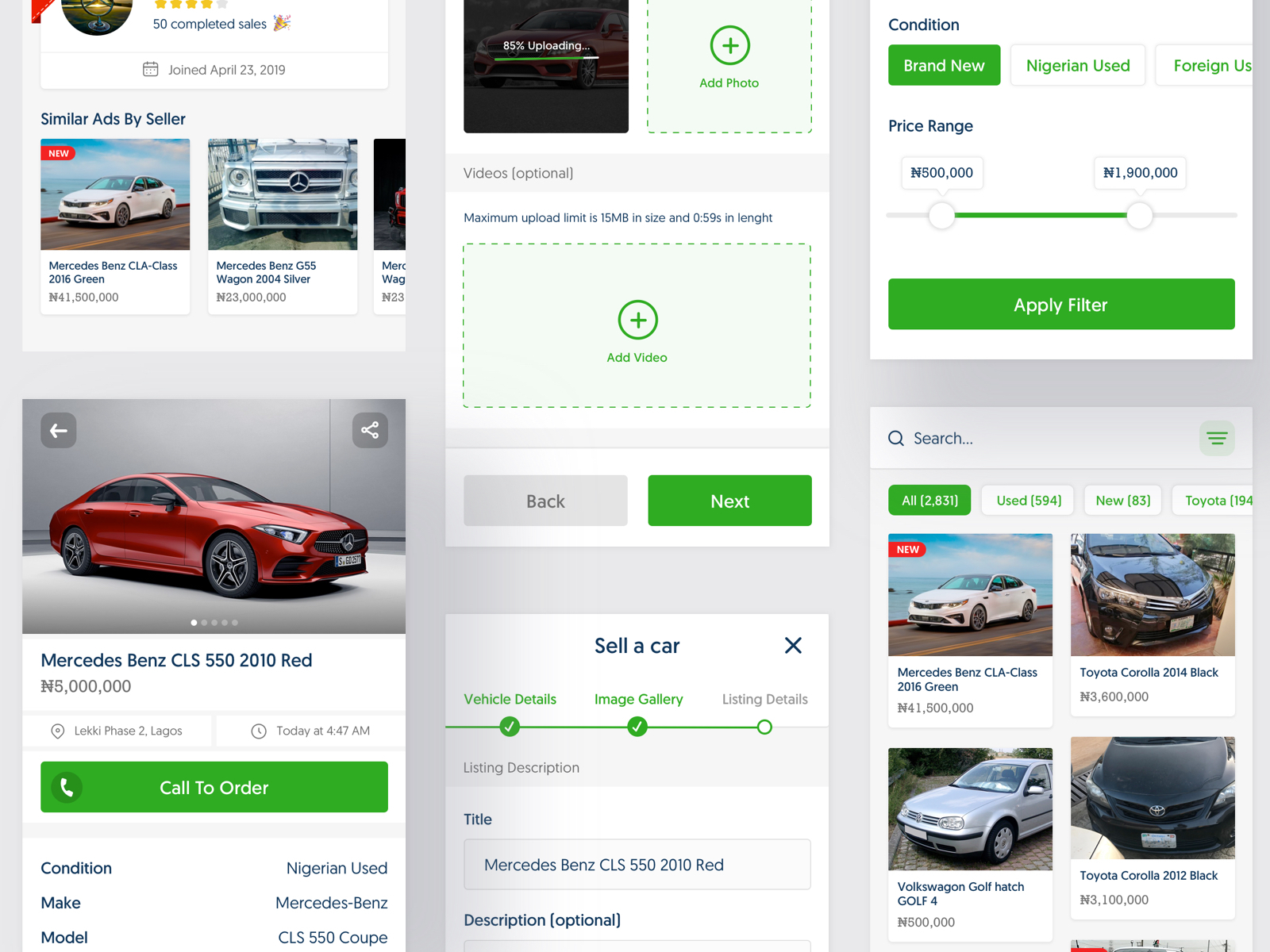This image depicts a zoomed-in screen capture of an online car sales platform. The screen has a light gray background with various white rectangles containing images and information about cars for sale. Due to the zoom, the top and bottom edges are cut off slightly. In the upper left corner, the user interface indicates that the seller has completed 50 sales since joining on April 23rd, 2019. Below, there is a section titled "Similar Ads by Seller," featuring listings such as a white 2016 Mercedes Benz CLA-Class. Further down, another listing for a red 2010 Mercedes Benz CL550 includes a noticeable "Call to Order" button with a white phone icon on the left.

On the lower part of the screen, an "Add Videos" section is visible with a "Next" button nearby. To the right, there is a section labeled "Sell Car," which contains areas for "Vehicle Details," "Image Gallery," and a status indicator showing that "Listing Details" have not yet been completed. This detailed layout provides a thorough view of the car listing process and available options on the platform.